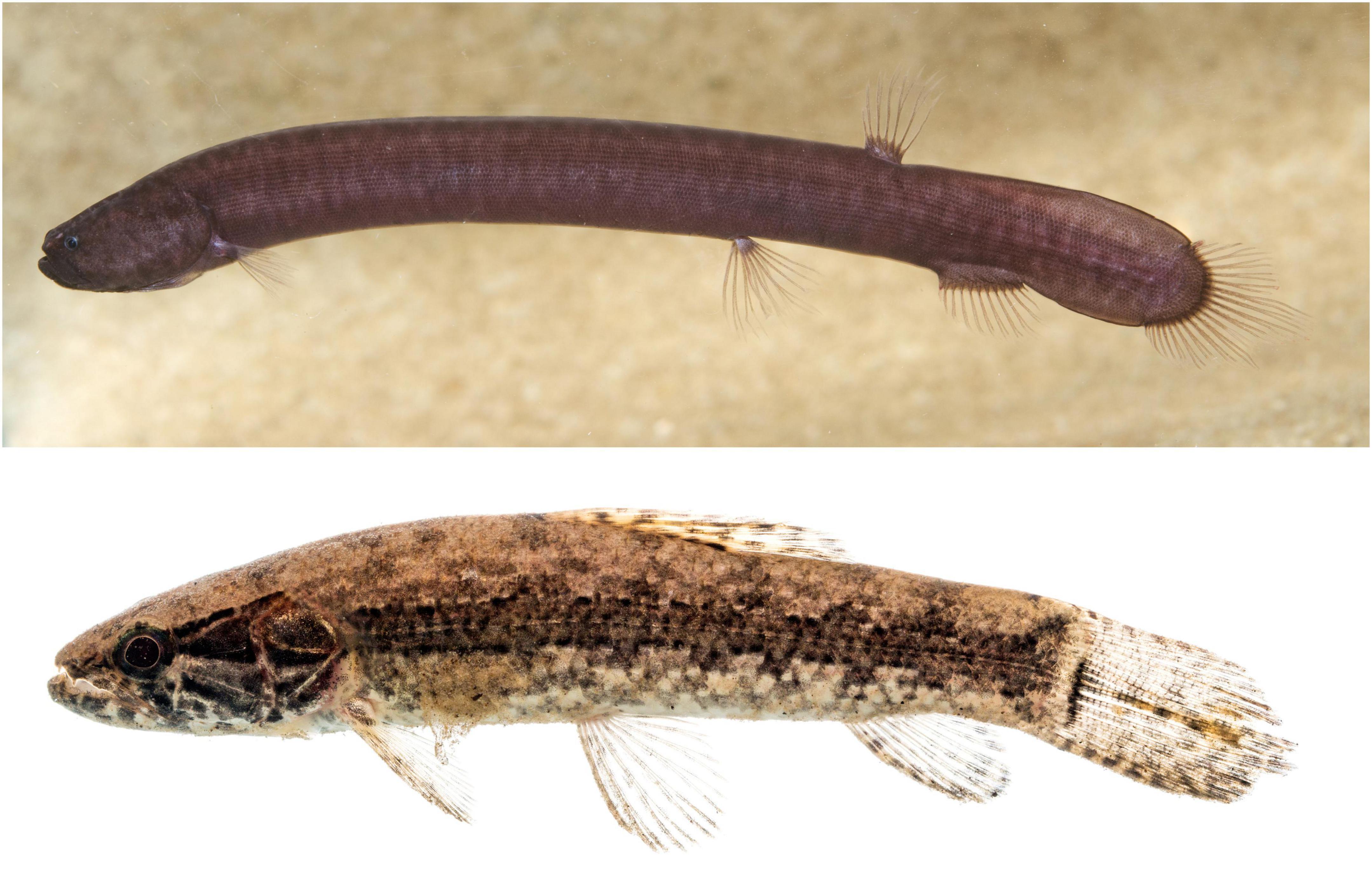The image consists of a set of two visual representations of fish, one above the other. The top image appears to be a photograph of a long, bizarre-looking fish with a reddish-brown to brown coloration, speckled with darker spots. It has a snake-like face and features several thin, translucent fins—a dorsal fin toward its tail, prominent pectoral fins near its gills, and another larger fin on its underside. The background of this photo is sandy and mottled, giving an underwater impression.

In contrast, the bottom image is an illustration or highly edited photograph with the background removed, leaving the fish on a plain white backdrop. This fish looks more conventional, resembling a minnow or a miniature salmon. It has a nondescript, mottled dark brown and light brown body with a prominent, darker lateral stripe. Its structure includes three fins on the bottom and one on the top, along with a swishy tail.

Both fish are depicted horizontally, implying they are swimming, and the images highlight the strong differences in appearance and possibly species, emphasizing the odd, almost prehistoric nature of the top fish compared to the more typical fish-like appearance of the bottom one.